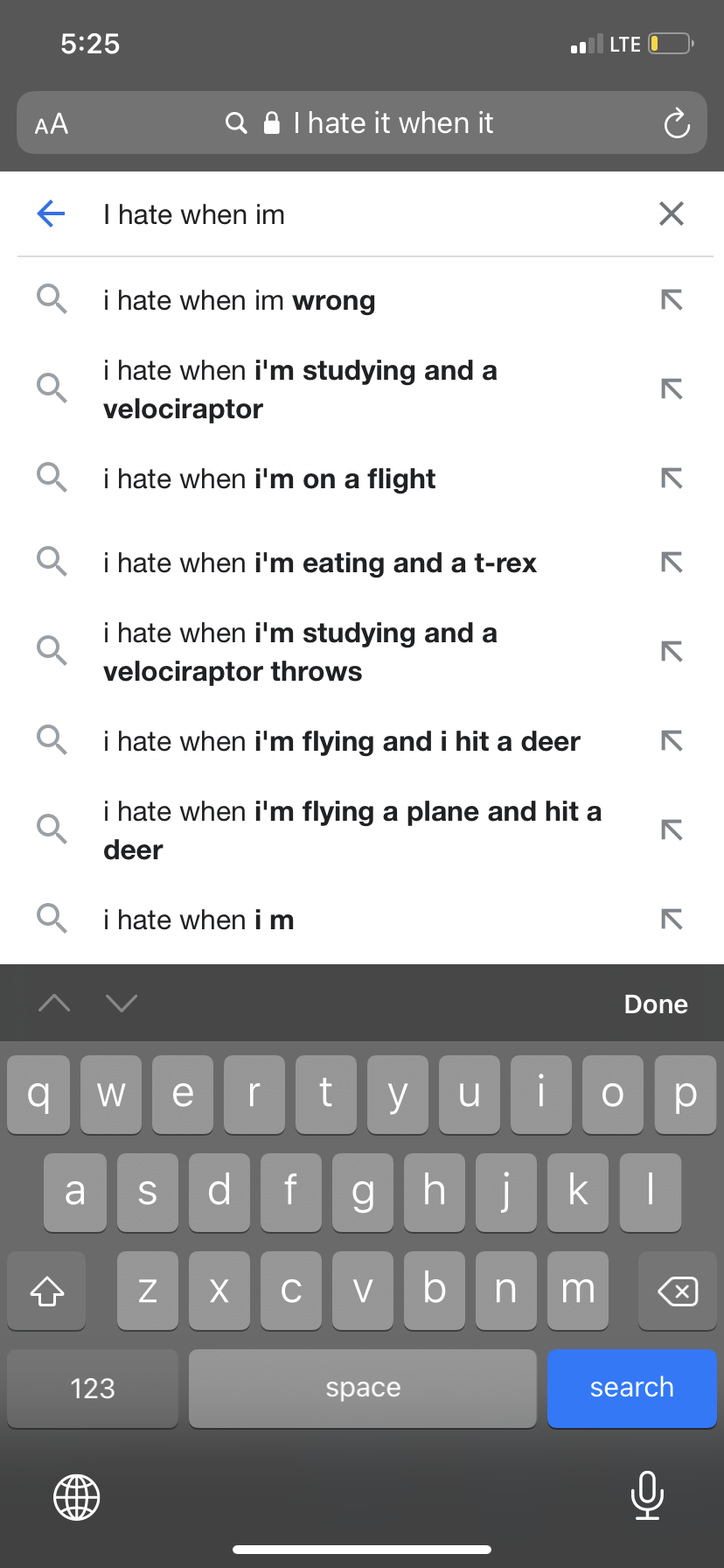The image features a smartphone screen with the time "5:25" displayed in the top left corner. In the top right corner, the phone shows cellular signal strength with two out of four bars for LTE, alongside a yellow, low battery symbol. Below the status icons, there is a block of text that reads, "I hate it when I'm wrong. I hate it when I'm studying and a velociraptor. I hate it when I'm on a flight. I hate it when I'm eating and a T-Rex. I hate it when I'm studying and a velociraptor throws. I hate it when I'm flying and I hit a deer. I hate it when I'm flying a plane and hit a deer. I hate it when I am." At the bottom of the screen, there is a gray keyboard. The main background of the image is white, with a light gray section at the top.